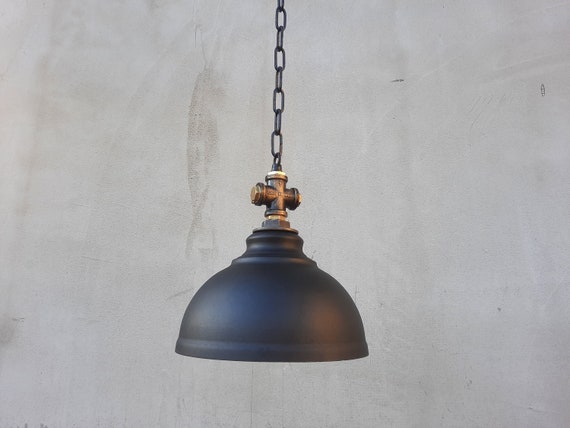The image showcases a modern, industrial-style hanging lamp suspended from a black chain. The lamp, which could be described as a blend between dark navy blue and black, features a metal, brass-colored crosspiece where the chain connects to the lamp. The fixture itself is shaped like an upside-down bowl or plunger, made from high-quality materials and displaying a well-crafted design. Attached to the base of the lamp is a noticeable metal switch with two protruding buttons. The background is predominantly a light gray and white hue, with subtle black and gray streaks that are only visible upon closer inspection. The overall scene lacks any illumination from the lamp, emphasizing its contemporary aesthetic against the empty background.